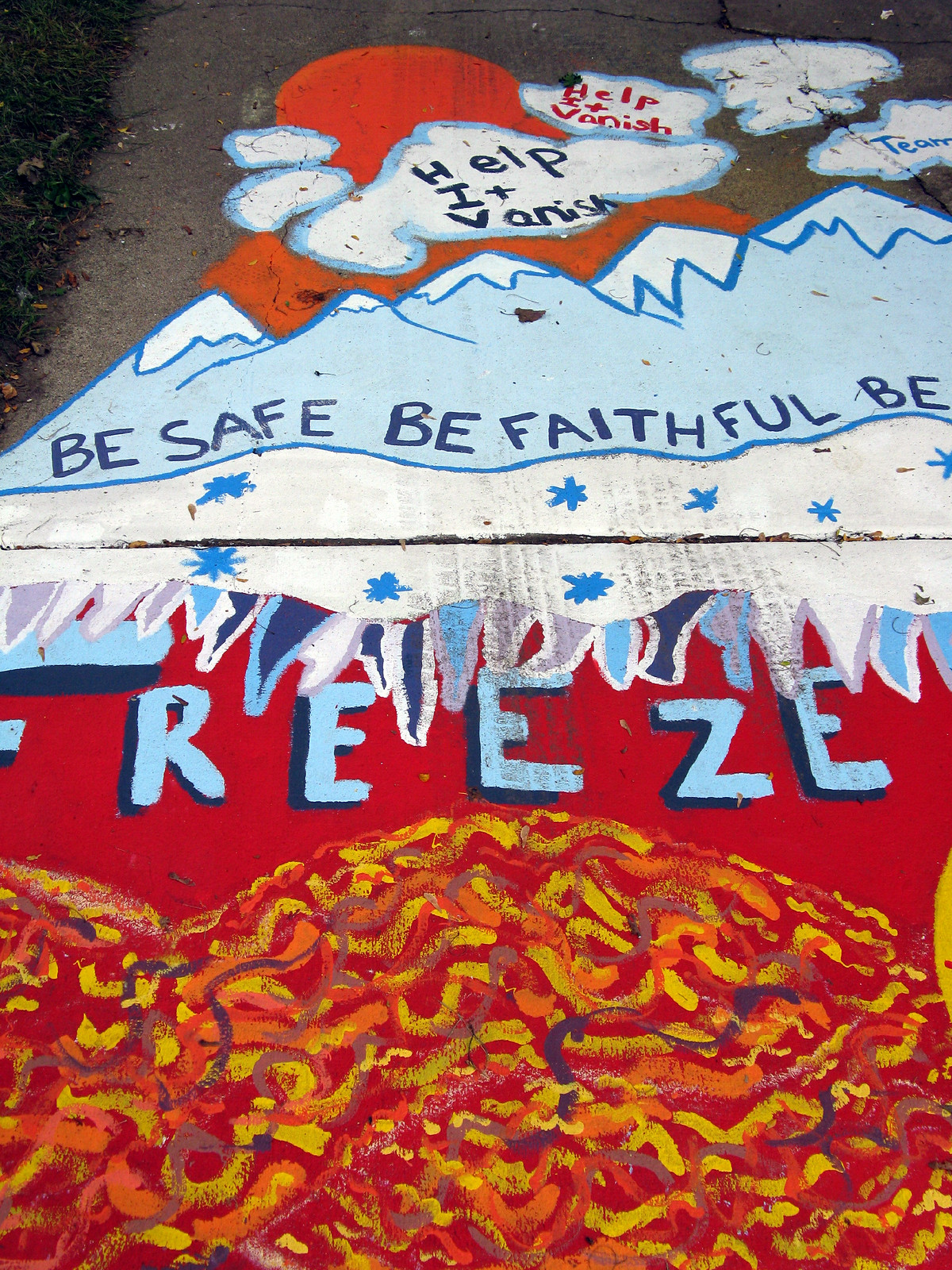The image showcases a detailed painted mural, possibly seen on a sidewalk, evoking a theme of safety and awareness with a vivid, multifaceted design. At the top, cloud-like shapes feature the phrase "Help It Vanish," with "HIV" creatively incorporated into the wording. In the central part of the mural, there are snow-capped, light blue mountains with the words "Be Safe, Be Faithful" painted in dark blue. Additionally, there's a partially obscured message in the same area. Below the mountains, snowflakes and the word "Freeze" are painted against a striking red background, reminiscent of lava. This area further transitions into a lower section filled with swirling lines in yellow, orange, and blue hues on the red surface, adding to the mural's dynamic and vibrant aesthetic.